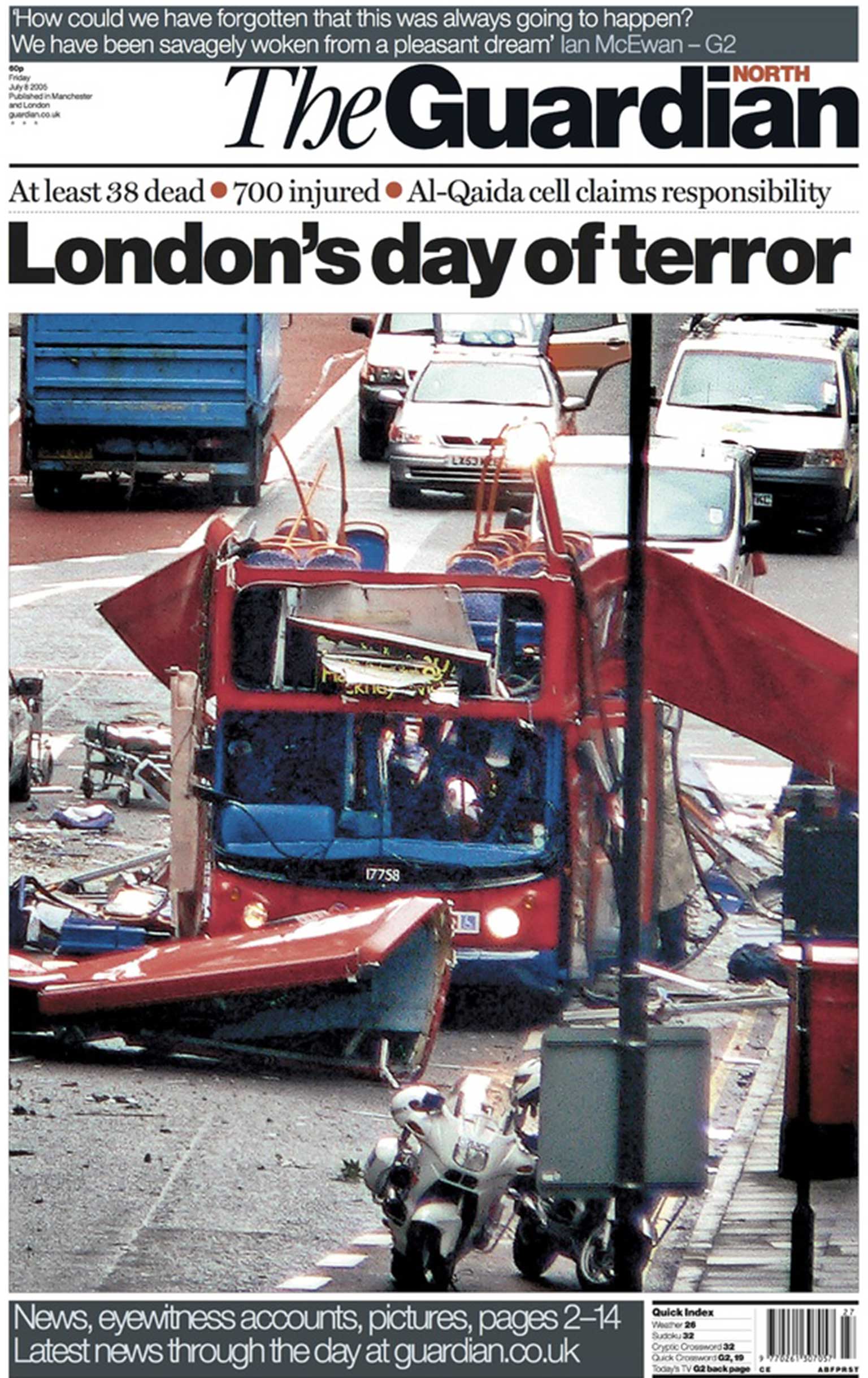This is the front page of The Guardian newspaper, prominently titled "The Guardian" in black font at the top right, with "North" positioned above it in red. Dominating the top section in a dark gray border is the quote, "How could we have forgotten this was always going to happen? We have been savagely woken from a pleasant dream," attributed to Ian McEwan, G2. Below the title, a stark headline in large black capital letters proclaims, "London's Day of Terror," followed by key details in black text and red circles listing, "At least 38 dead," "700 injured," and "Al-Qaeda cell claims responsibility."

An image beneath the headline reveals the aftermath of a devastating incident involving a red double-decker bus that appears to have been bombed. The roof is completely blown off, exposing blue seats on the top deck amidst a chaotic scene of twisted metal fragments and surrounding debris. Other vehicles, including a blue truck and several cars and motorcycles, are halted around the wreckage on a gray street lined with debris and a lone pole.

At the bottom in white text on a gray background, the page offers more information: "News, eyewitness accounts, pictures, pages 2 through 14," and directs readers to "guardian.co.uk" for the latest updates. A barcode sits at the bottom right corner, completing the layout of this somber yet informative cover.